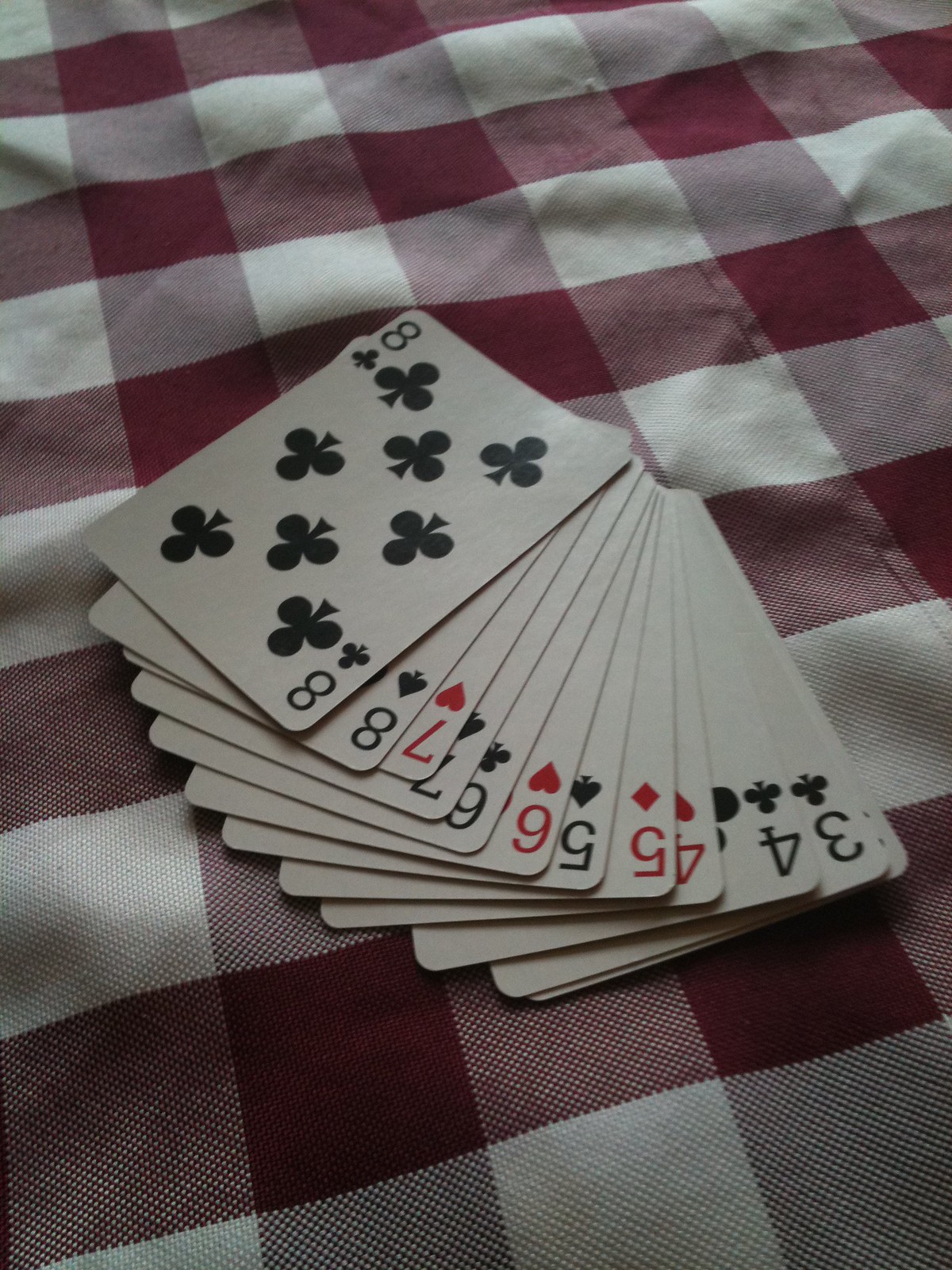The image displays a detailed arrangement of playing cards from a deck, each adorned with various patterns. These cards are meticulously spread out in a fan-shaped formation, reminiscent of how one might hold a hand during a card game. They are laid across a red and white checkered tablecloth that covers the entire table.

In the fan arrangement, the card on top features the black cloverleaf symbol, commonly known as the clubs suit, and is marked with the number eight, indicating its rank. Following this top card, the remaining cards are visible in descending numerical order: seven, six, five, four, three, and onwards, with each number appearing twice — two eights, two sevens, and so on, down to the number one.

The repetition of numbers and the precise alignment of the cards in this display highlights a sense of order and symmetry, contributing to a visually appealing and organized presentation. Each card is clearly visible, showcasing the patterns and numeric sequence effectively against the contrasting backdrop of the checkered tablecloth.